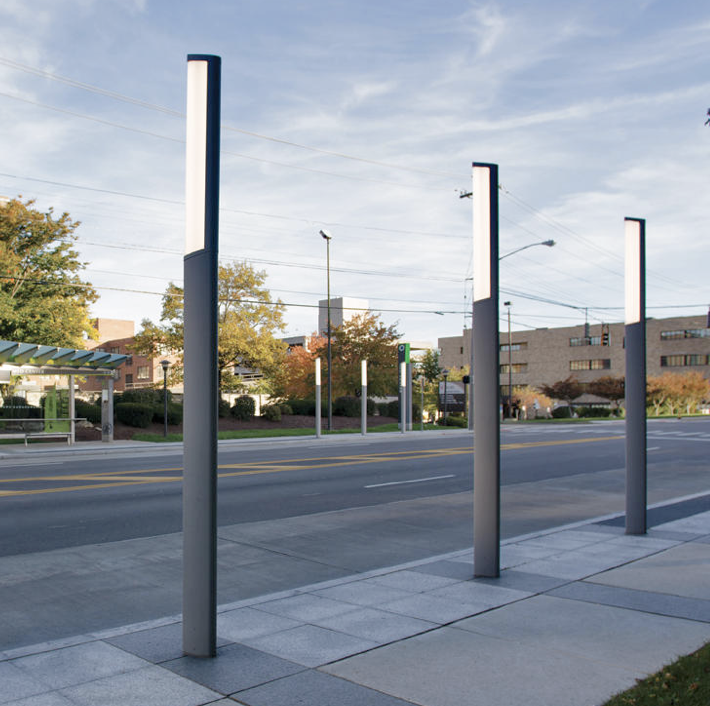This image depicts a daytime scene in a somewhat urban setting with low-rise buildings, potentially public institutions like a hospital or university, in the background. In the foreground, we are positioned just off the sidewalk, which extends about two blocks wide, moving in a direction that could be described as two o'clock. The street next to the sidewalk features three lanes: two heading right and one heading left. Prominently visible are three modern streetlights, resembling vertical gray tubes of uniform width, standing a couple of stories high, with light bars at the top, possibly solar-powered and seemingly glowing despite the sunlight. 

Across the street, a glass-enclosed bus stop with a wavy silver roof can be seen. The sky is partly cloudy with wispy white clouds stretching from left to right. The area has a warmer climate, as suggested by lush, green-leafed oak trees that dot the landscape, contributing to the overall serene yet functional atmosphere of the scene. The streets and sidewalks appear relatively empty, emphasizing the tranquil and orderly nature of this public space.